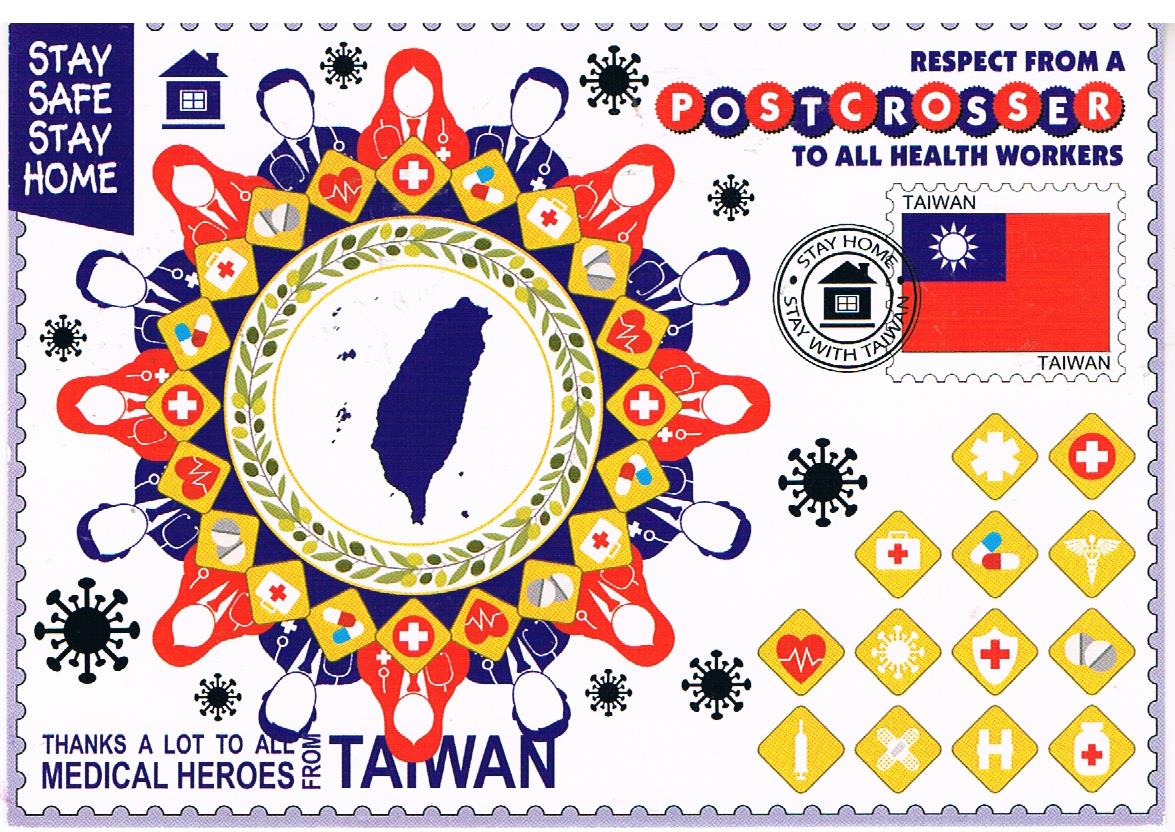The image is a vibrant, postcard-like design commemorating the health workers of Taiwan, prominently styled with the look of a postage stamp featuring serrated edges and a thin, light purple border. Set against a detailed white background, the primary colors—blue, red, yellow, and light blue—stand out vividly. 

At the top left, a blue angled bar with white letters reads "Stay Safe, Stay Home." Beneath this, there is a small icon of a blue house. Moving down the left edge, there are small black symbols representing the COVID-19 virus. Adjacent to this, blue letters spell out "Thanks a lot to all," followed by "MEDICAL HEROES" in larger font, and the note "from Taiwan" in bold text.

The center of the postcard features a detailed circular table-like design with alternating red and blue figures of healthcare professionals—eight men in blue with ties and stethoscopes, and eight women in red with shoulder-length red hair and stethoscopes—giving the appearance of a mandala. Surrounding this central design are yellow squares containing various medical symbols, such as the Red Cross, pills, first-aid kits, capsules, and hearts. Encircling the healthcare professionals is an inner floral-like ring, with an illustrated map of Taiwan within the center.

In the top right corner, "Respect from a post crosser to all health workers" is written, with "POSTCROSSER" prominently highlighted in an alternating red and blue circular pattern with white letters inside. Directly below this, a stylized stamp displays the Taiwanese flag and a postmarked message that reads, "Stay home, stay with Taiwan," alongside another house icon.

The lower right corner mirrors the medical symbols from the center, arranged in rows within yellow squares, totaling thirteen symbols. Scattered around the lower portion are additional small black representations of the COVID-19 virus.

Overall, the image serves as a colorful, intricate tribute to the medical heroes of Taiwan, rich with symbols of healthcare and solidarity.